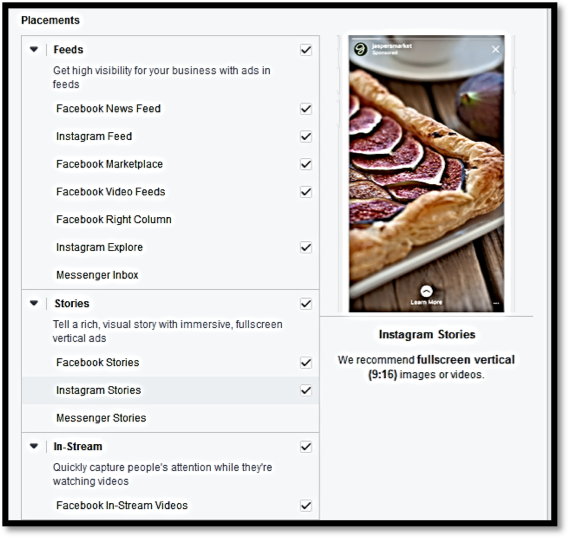The image is a screenshot of an Instagram story showcasing an advertising management interface with details about various ad placements. The top left corner of the screenshot features the word "Placements" on a white background with black text, enclosed in a rectangular box divided into three sections. Below "Placements," the first section is labeled "Feeds," which is a dropdown menu that is currently expanded. It displays the message: "Get high visibility for your business with ads in feeds" and lists multiple options for ad placements, each accompanied by a clickable tick box. The options include Facebook News Feed, Instagram Feed, Facebook Marketplace, Facebook Video Feeds, Facebook Right Column, Instagram Explorer, and Messenger Inbox.

The second section, titled "Stories," also features a dropdown menu that is expanded to reveal the message: "Tell a rich visual story with immersive full screen vertical ads." The available ad placement options here, all with clickable tick boxes, are Facebook Stories, Instagram Stories, and Messenger Stories.

The final section, "In Stream," highlights the ability to "quickly capture people's attention while they're watching videos," with ad placement options specifically for Facebook In Stream Videos, also marked with a clickable tick box.

On the right-hand side of the screenshot, there's an image of a savory pastry, suggesting the type of content that might be used in the ads. The Instagram story interface is evident from the username and progress bars at the top, indicating how many stories the user has posted.